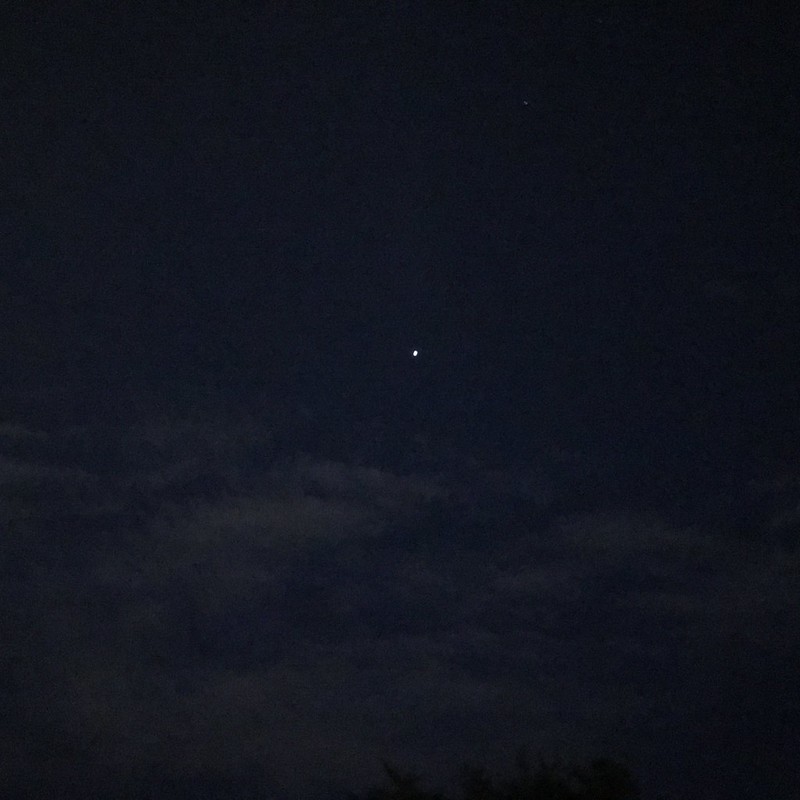This photograph captures a tranquil night sky dominated by a deep black canvas. At first glance, the image appears to be a simple square of plain black, but a closer inspection reveals its subtleties. Near the lower portion of the photograph, you can see dusty gray clouds softly hanging in the sky, adding an element of texture. The sky is punctuated by a brilliant white dot situated near the center of the image, likely representing a luminous star or perhaps a planet, given its significant size compared to other celestial objects. Just above this bright focal point lies a smaller, dimmer star. The clouds' presence, along with their grayish hue, suggests this scene was captured shortly after sunset. Additionally, the very bottom of the photo hints at the tops of trees, grounding this celestial view in an earthly context.